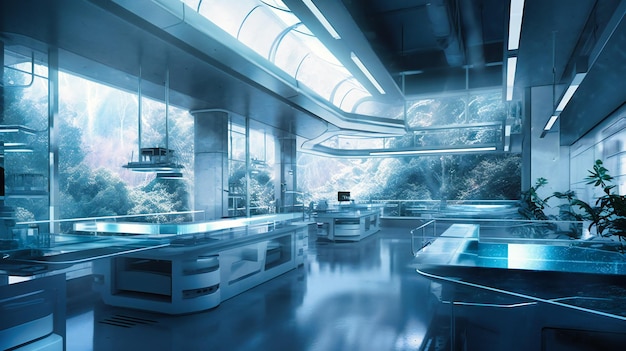This image is a landscape-oriented photograph of a spacious, futuristic room that blends elements of a living room, kitchen, and possibly even a workspace or restaurant. It is bathed in abundant natural light from very tall, high glass windows that provide a view of a lush, possibly tropical forest, enveloping the structure in greenery. Three large islands with glass tops and silver bases dominate the room, giving it a sleek and modern appearance. The room’s overall color scheme is muted, primarily showcasing shades of gray, white, and a subtle muted blue, all illuminated by bright, fluorescent overhead lighting, which runs the length of the ceiling and adds a glowing, sterile ambiance. The minimalistic and clean design is accentuated by the absence of people and the sparsely placed green plants along the right-hand side, contributing to a sense of serenity and sophistication.